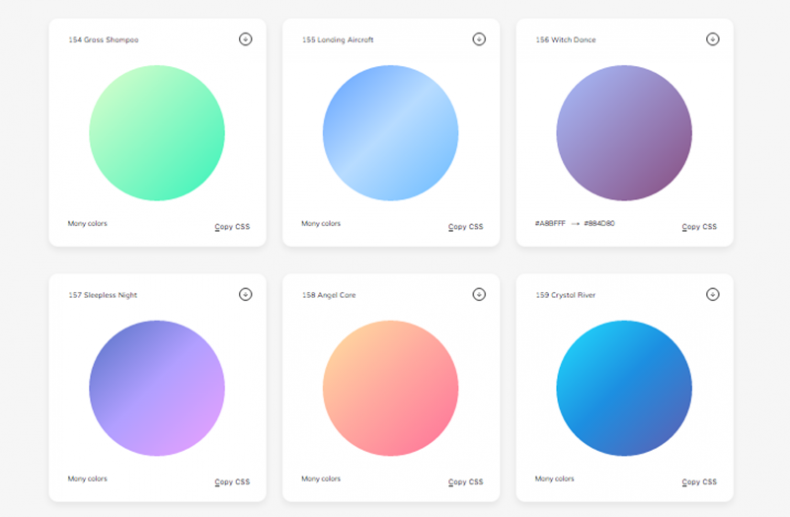The image features a light gray background that is thicker on the left and right sides compared to the top and bottom. Within this background are six evenly spaced white squares arranged in two rows of three. Each square contains a colored circle, with a thin gray line separating each square from the others. 

- The first square at the top row contains a green circle, numbered 154, and is labeled "Grass Shampoo." Below this, the text reads "Many Colors" and "Copy CSS."
- The second square features a blue circle, numbered 155, and is titled "Landing Aircraft." Similar to the first, it has "Many Colors" and "Copy CSS" at the bottom.
- The third square in the top row showcases an ombre purple circle, transitioning from lighter at the top to darker at the bottom diagonally. It is numbered 156 and called "Which Stands." This also includes the labels "Many Colors" and "Copy CSS."

On the bottom row:
- The first square has a purple circle with a gradient fading from darker to lighter purple diagonally. It is numbered 157 and named "Sleepless Nights," accompanied by the same "Many Colors" and "Copy CSS" text.
- The second square displays a peach circle that transitions to a darker melon color. Numbered 158, it is titled "Angel Core," including the "Many Colors" and "Copy CSS" text at the bottom.
- The third square features a blue circle that fades from a lighter blue to a darker blue, numbered 159 and labeled "Crystal River." It also contains the "Many Colors" and "Copy CSS" text at the bottom.

This detailed arrangement provides a clear depiction of colors and names along with their CSS copying options.